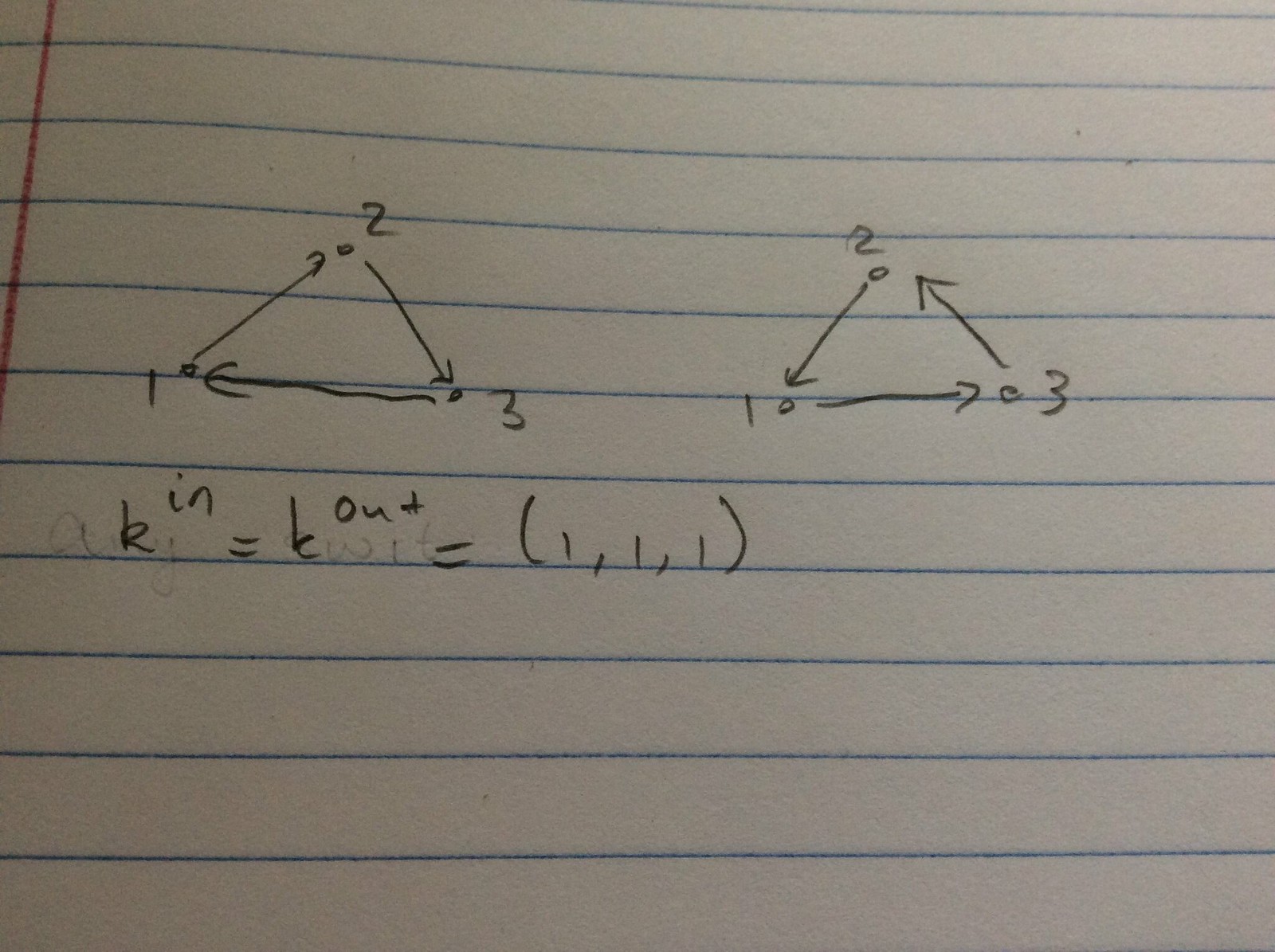The image depicts a piece of lined notebook paper adorned with drawings and notations made using a very dark instrument, possibly a mechanical pencil or a black pen. The sheet features two distinct triangles, both annotated with directional arrows and numbers.

On the left side, the first triangle is labeled with points 1, 2, and 3. Point 1 is located at the bottom corner with an arrow pointing upwards to point 2 at the center. From point 2, an arrow points downwards to point 3 at the bottom right corner, and another arrow returns from point 3 to point 1, completing the cycle.

On the right side, the second triangle differs in its directional flow despite having similar points numbered 1, 2, and 3. Here, point 1 starts at the bottom left corner, with an arrow extending along the bottom line to point 3 at the bottom right. Point 3 has an arrow pointing upwards to point 2 in the center. Finally, point 2 directs an arrow back down to point 1, forming a flow opposite to the triangle on the left.

Additionally, there is a mathematical formula noted at the top of the page. It reads: "R^I, N = T_out = (1, 1, 1)," indicating a relationship or result that is part of the broader context of the image, perhaps hinting at a problem or proof in geometry or algebra.